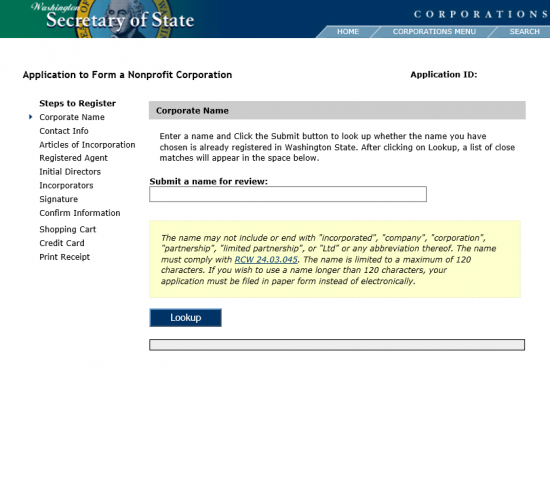This is a detailed caption for the given image:

"The image depicts a screenshot taken from a desktop, showcasing an official webpage titled 'Washington Secretary of State.' In the top left-hand corner, the title 'Washington Secretary of State' is prominently displayed next to a background image of George Washington. On the top right-hand corner, the title 'Corporations' is visible with three clickable buttons underneath: 'Home,' 'Corporations Menu,' and 'Search.' 

Centrally located on the webpage, there is an interactive section where users can submit a name for review. Above this section, a description instructs users to 'Enter a name and click the Submit button to look up whether the name you have chosen is already registered in Washington State. After clicking Lookup, a list of close matches will appear in the space below.' At the bottom of this section, there is a prominently displayed blue button labeled 'Lookup.'

To the left side of the webpage, there is a vertical list of steps required for the registration process. The list reads as follows: 'Corporate Name,' 'Contact Info,' 'Articles of Incorporation,' 'Agent,' 'Initial Directors,' 'Incorporators,' 'Signature,' 'Confirm Information,' 'Shopping Cart,' 'Credit Card,' and finally, 'Print Receipt.'"